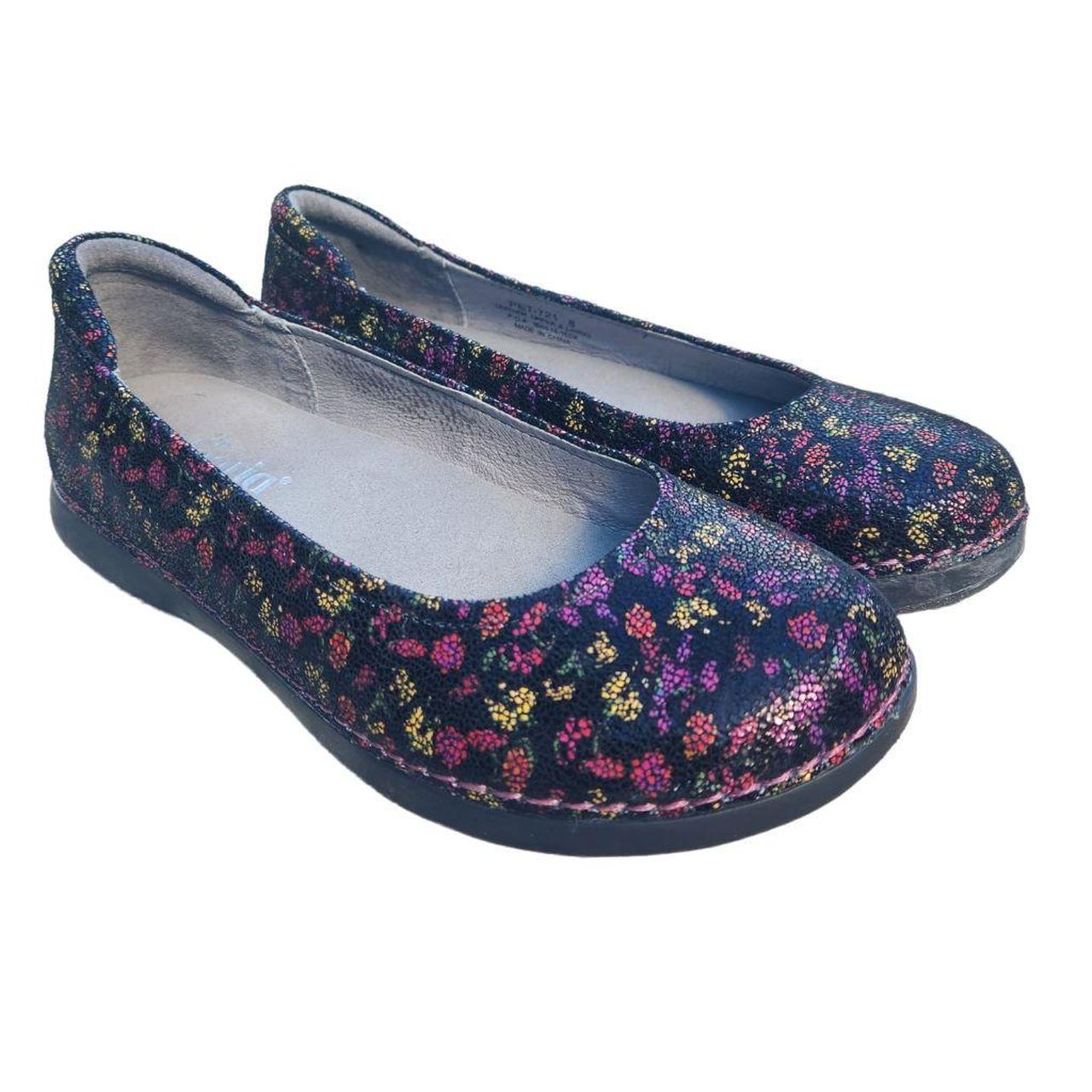The close-up image features a pair of women's low-cut, slip-on loafers, which bear a resemblance to traditional Japanese or Chinese slippers. These shoes are crafted from a synthetic material and have a distinct black rubber sole. The upper part of the shoes showcases an intricate floral pattern set against a black background. This pattern consists of small, circular dots in vibrant colors such as red, purple, pink, orange, yellow, and even some green that resemble clusters of berries or flowers. The interior of the shoes is lined with a soft, gray material that appears quite comfortable. There is silver writing on the heel part of the sole, though it is not legible. The soles and tops are securely stitched, and despite showing some signs of wear, the shoes are still in good condition.